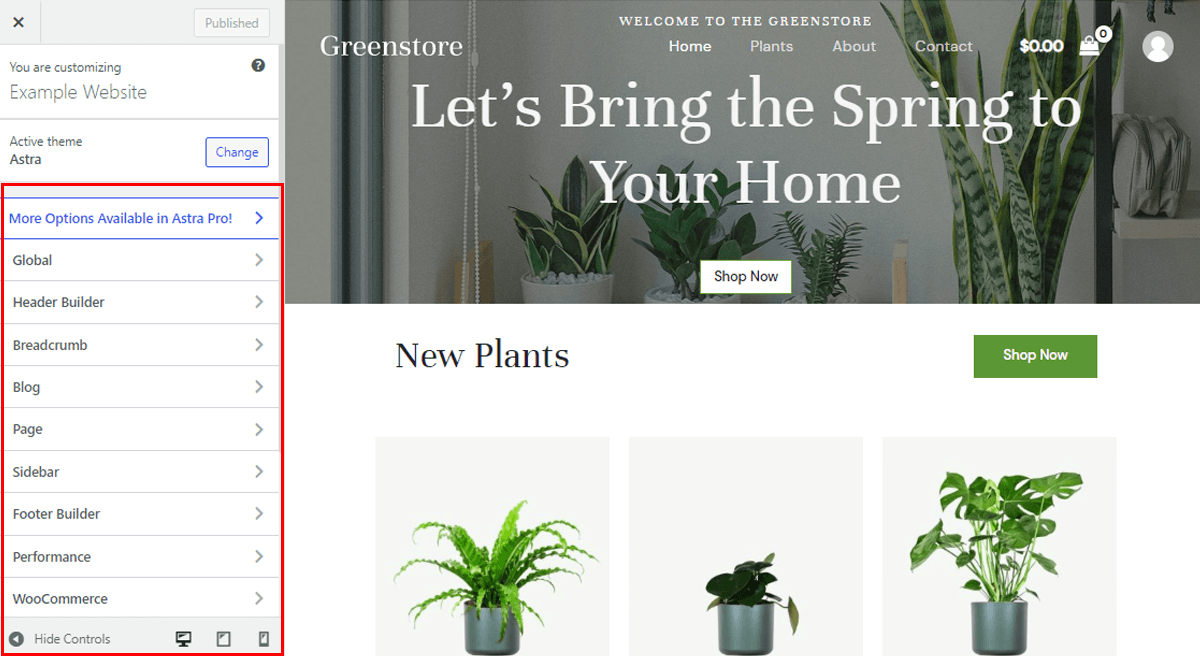Detailed Caption: 

The image depicts a web page for a store named "Green Store" that specializes in selling plants. The web page is still under construction, as evidenced by the customization interface open on the left. On the far left, a vertical panel is dedicated to website customization options. At the top of this panel, a gray bar contains an "X" icon on the left and a grayed-out "Published" button on the right. Below this, the background turns white and features the heading "You are customizing," with "Example Website" prominently displayed in larger letters. To the top right within this pane, a dark dot with a question mark provides further assistance.

Continuing down this pane, the background remains white and displays "Active Theme: Astra" alongside a gray rectangular "Change" button. A red outline highlights the next section, with a blue header stating "More Options Available in Astra Pro," accompanied by a right-facing caret icon. Below this, nine rows list various customization options, each flanked by a right-facing caret. These options, written in dark gray, include: Global, Header Builder, Breadcrumb, Blog, Page, Sidebar, Footer Builder, Performance, and WooCommerce. At the bottom of the red-outlined rectangle, a gray bar reads "Hide Controls," with icons flanking either side.

To the right of this customization panel is a preview of the web page. At the top, a gray banner features a subtly grayed-out background image of plants in a room, overlaid with the text "Let's Bring the Spring to Your Home" and a white rectangular "Shop Now" button. Above this banner, in tiny white letters, it reads "Welcome to the Green Store." Below this greeting, the larger header "Green Store" appears on the left, with a navigation menu on the right listing "Home," "Plants," "About," and "Contact," followed by a "Zero Dollars" indicator next to a shopping bag and a person icon, signifying the account section.

The main area of the web page showcases three square photographs of plants at the bottom, each set against a gray background. Each plant is housed in a black pot with either lush green leaves or, in the case of the middle plant, shorter, darker leaves. Above these images, the section title "New Plants" is displayed in large dark letters, adjacent to a green rectangular "Shop Now" button in white.